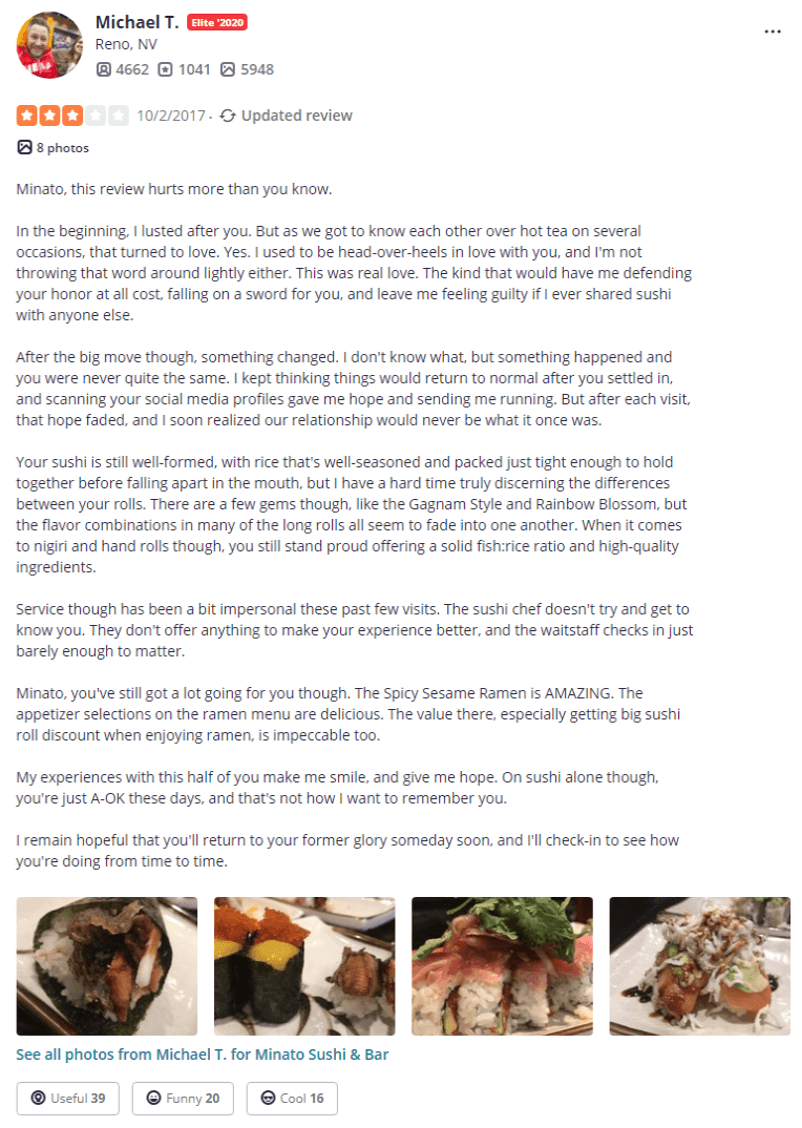**Detailed Caption:**

This image showcases a screenshot of a review written by a user named Michael T on a website. In the top left-hand corner, there is a circular profile picture of a man with brown hair, a brown goatee, and a red shirt. To the right of the profile picture, the name "Michael T" is displayed in bold black letters. Beneath his name, "Reno, NV" is written in gray letters.

Moving further down, the review shows a three-star rating highlighted in orange, with the date "10-20-2017" beside it. To the right, there is a refresh button accompanied by the text "Update Your Review." 

Below, on the left side, there is an icon indicating photos, with the text "8 photos" in black next to it. The body of the review reads:

"Monado, this review hurts more than you know. In the beginning, I lusted after you, but as we got to know each other over hot tea on several occasions, that turned to love. Yes, I used to be head over heels in love with you, and I'm not throwing that word around lightly either. This was real love, the kind that would have me defending your honor at all costs, falling on a sword for you, and feeling guilty if I ever shared sushi with anyone else. After the big move, though, something changed. I don't know what, but something happened and you were never quite the same. I kept thinking things would return to normal after you settled in, and scanning your social media profiles gave me hope and sent me running, but after each visit, that hope faded, and I soon realized our relationship would never be what it once was.

Your sushi is still well-formed with rice that's well-seasoned and packed just tight enough to hold together before falling apart in the mouth, but I have a hard time truly discerning the differences between your rolls. There are a few gems though, like the Gan Nam Style and Rainbow Blossom, but the flavor combinations in many of the long rolls all seem to fade into one another. When it comes to the nigiri and hand rolls though, you still stand proud, offering a solid fish-to-rice ratio and high-quality ingredients. 

However, service has been a bit impersonal these past few visits. The sushi chef doesn't try to get to know you. They don't offer anything to make your experience better, and the waitstaff checks in just barely enough to matter. Monado, you've still got a lot going for you though. The spicy sesame ramen is amazing. The appetizer selection on the ramen menu is delicious. The value, especially getting a big sushi roll discount when enjoying ramen, is impeccable too. My experiences with this half of you make me smile and give me hope. On sushi alone though, you're just okay these days, and that's not how I want to remember you. I remain hopeful that you'll return to your former glory someday soon, and I'll check in to see how you're doing from time to time."

At the bottom of the page, there are four thumbnail images of various sushi dishes.